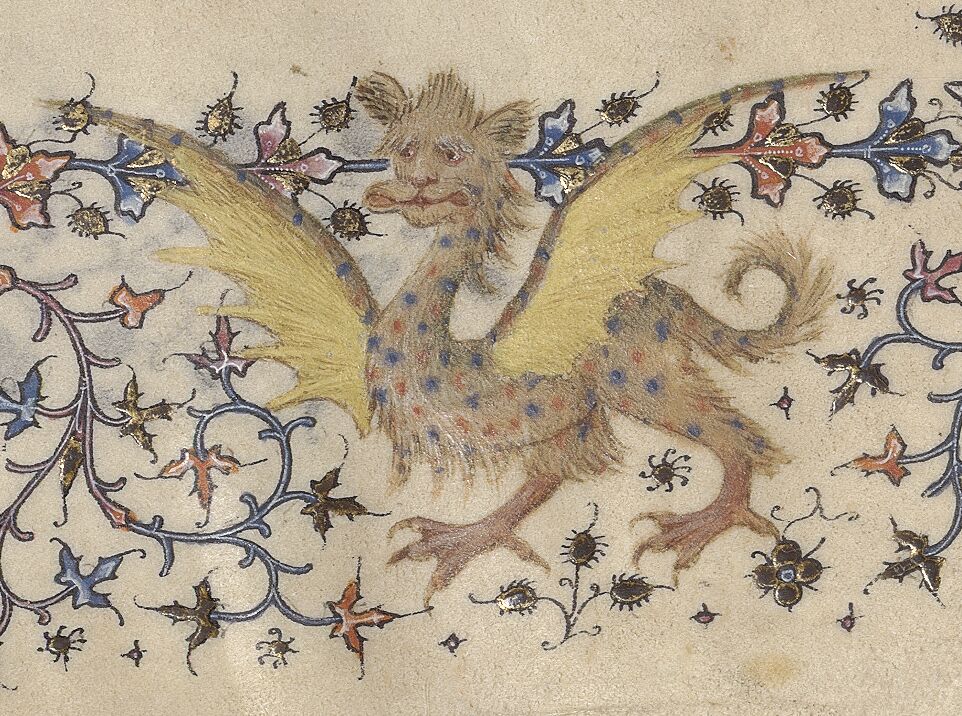The image depicts a seemingly ancient and worn embroidered fabric illustrating a fantastical mythical creature that blends characteristics of various animals. This central figure, a blend of dragon and griffin, features a fur-covered body adorned with blue and orange dots stretching from its long, giraffe-like neck to its curly, dog-like tail. The creature's face, framed by thick bushy eyebrows, displays human-like features: a large mouth, prominent ears, and an expressive visage. It sports light yellow dragon wings, bird-like taloned feet, and a body covered in wispy hair. Surrounding the creature are intricate decorations of tree-like vines and spear-like structures, interspersed with blue, brown, and red floral and seed pod motifs, set against a light brown background. The overall scene evokes a medieval or mythological feel, showcasing an intricate interplay of colors and detailed embroidery. There are no visible texts or signatures on the image.